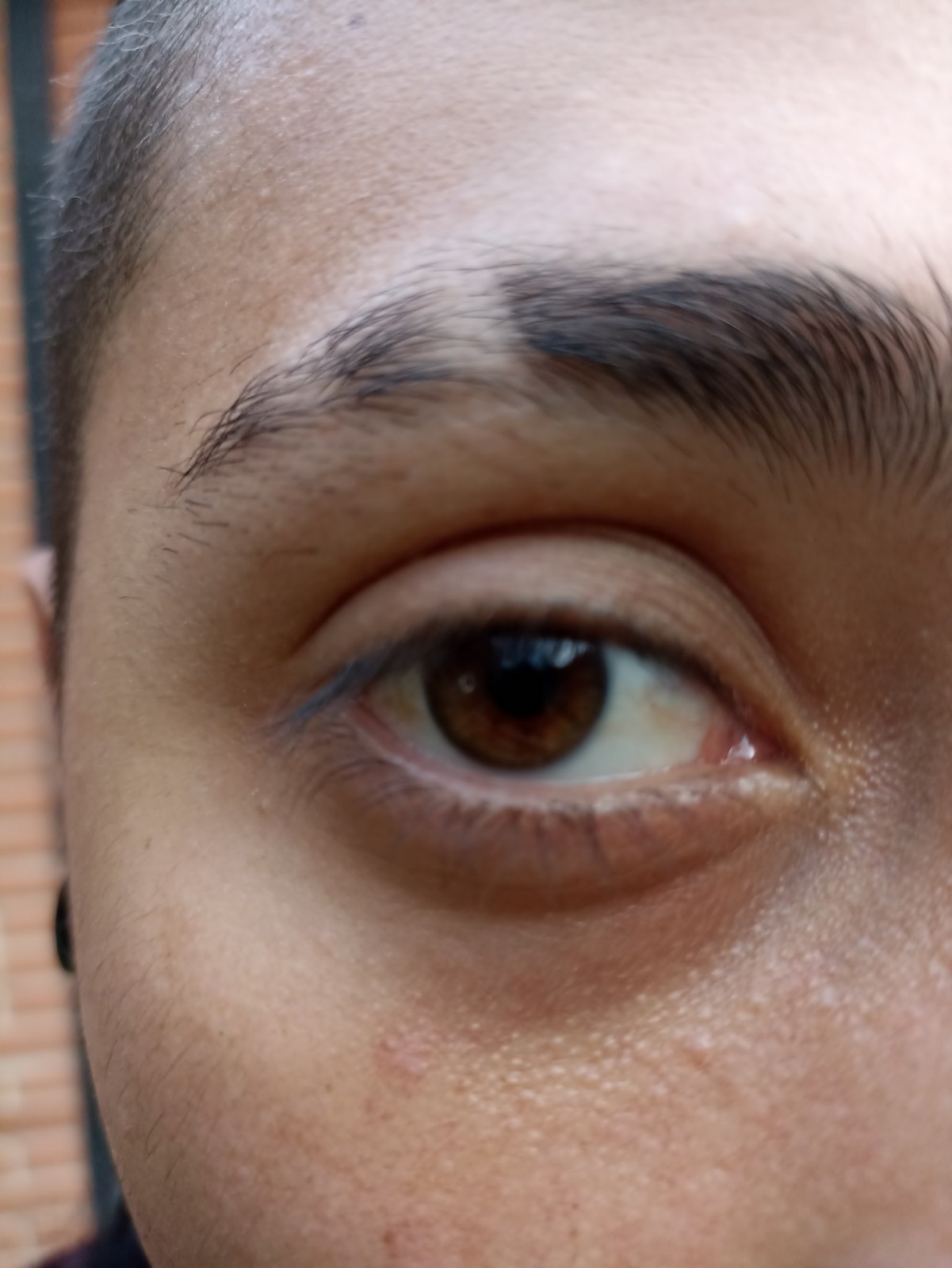This detailed close-up photograph captures the right eye of a person, framed by short black hair and a background that remains mostly indistinct. From our perspective, it’s the left eye, and its dark brown color is distinctly highlighted alongside the intricate network of blood vessels noticeable on the sclera. The eyebrow arches gracefully with a few visible gaps, suggesting a deliberate grooming style, while appearing thick due to the proximity of the shot. The eye is central to the image, bordered by light brown skin that exhibits a slightly tan complexion. A flat against-the-head ear is faintly visible on the left edge, adorned with what seems to be a small black earring or stud. The upper cheek blends into the hairline, completing the intimate portrayal of the person's eye and a portion of their face. The dark pupil contrasts starkly against the brown iris, adding depth to the eye's gaze. The photograph showcases the fine details of the face, making the eyeball and surrounding area the primary focus.